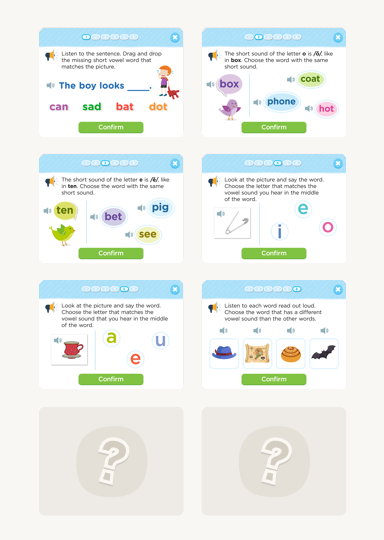This detailed illustration depicts an educational web page designed for teaching vowel sounds through interactive fill-in-the-blank exercises. Each interactive element is centered on a gray background, with a distinctive cyan blue bezel at the top. Small numbered buttons, from 1 to 6, are lined across the top, with two additional buttons marked by question marks at the bottom.

### Descriptive Breakdown:

1. **Interactive Panel 1:**
    - **Instruction:** "Listen to the sentence, drag and drop the missing short vowel word that matches the picture."
    - **Visual Content:** An image of a red-haired child—either a boy or girl—holding a red stuffed animal. The child wears a red undershirt, a purple overshirt, black shorts, and blue shoes.
    - **Audio Cues:** Adjacent to a blue megaphone icon, it repeats the instruction.
    - **Interactive Elements:** A sound icon and selectable words "can," "sad," "bad," and "not" appear below the phrase, "The boy looks sad," underlined in blue.

2. **Interactive Panel 2:**
    - **Instruction:** "The short sound of the letter 'O' is /ɒ/ as in 'box.' Choose the word with the same short sound."
    - **Visual Content:** A purple bird with dark purple wings and a thought bubble saying "box."
    - **Audio Cues:** A sound icon in a cyan circle.
    - **Interactive Elements:** Select words from circles labeled "phone" (cyan), "coat" (light green), and "hot" (pink).

3. **Interactive Panel 3:**
    - **Instruction:** "The short sound of the letter 'E' is /e/, as in 'ten.' Choose the word with the same short sound."
    - **Visual Content:** A bird with light green and dark green features and orange feet.
    - **Audio Cues:** A sound icon in a green circle.
    - **Interactive Elements:** Select words from circles labeled "ten" (light green), "pen" (purple), "pig" (cyan), and "see" (yellow).

4. **Interactive Panel 4:**
    - **Instruction:** "Look at the picture and say the word. Choose the letter that matches the vowel sound you hear in the middle of the word."
    - **Visual Content:** A gray, open clothespin.
    - **Audio Cues:** A sound icon nearby.
    - **Interactive Elements:** Select letters from circles labeled "i" (cyan), "e" (cyan), and "o" (cyan, hot pink).

5. **Interactive Panel 5:**
    - **Instruction:** "Look at the picture and say the word. Choose the letter that matches the vowel sound you hear in the middle of the word."
    - **Visual Content:** A red teacup with gray dots, a white interior, and a white saucer.
    - **Audio Cues:** A sound icon next to it.
    - **Interactive Elements:** Select letters from circles labeled "a" (green), "e" (orange), and "u" (blue).

6. **Interactive Panel 6:**
    - **Instruction:** "Listen to each word read out loud. Choose the word that has a different vowel sound than the other words."
    - **Visual Content:** Four objects – a blue hat with a red band, a gray map, an orange-and-brown-striped beehive, and a black bat.
    - **Audio Cues:** Sound icons above each object.
    - **Interactive Elements:** Identify the word with a different vowel sound.

The two additional, yet locked, panels are shaded in dark gray with darker gray question marks bordered in white, hinting at more advanced exercises.